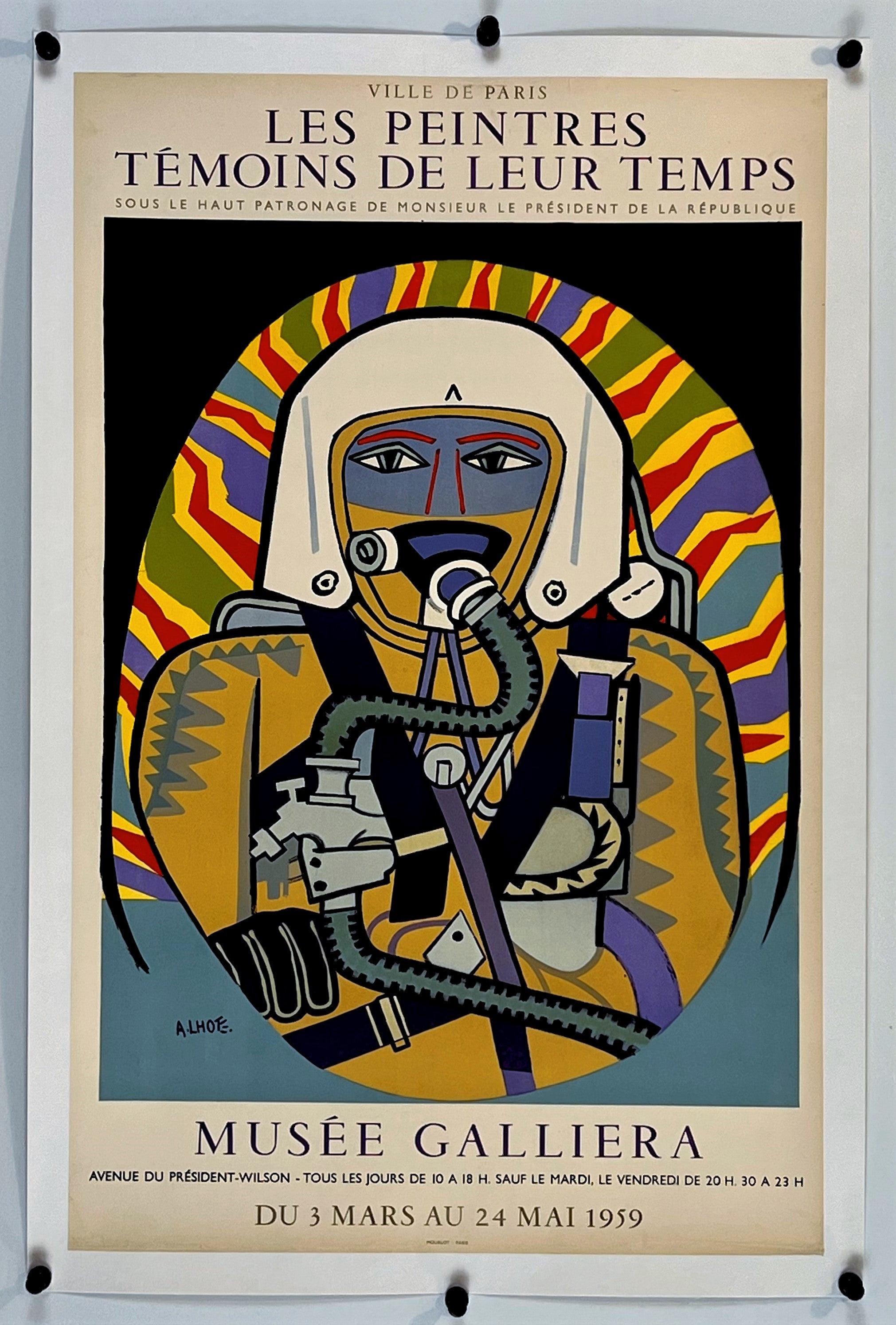This image depicts an abstract theater poster pinned to a bulletin board with six black pins, three securing the top and three anchoring the bottom. The poster artwork features an abstract portrait of a person adorned with what appears to be a pilot's helmet, complete with an oxygen tube extending from it. The figure's right hand, covered by a glove, is visible. The face is partially obscured by a blue mask that allows the person's striking green and black eyes to be seen, complemented by vivid red eyebrows. Surrounding the figure, radiant lines of blue, olive green, red, and yellow fan out dramatically from the background. The text on the poster is in French, suggesting this could be related to a French theater production.